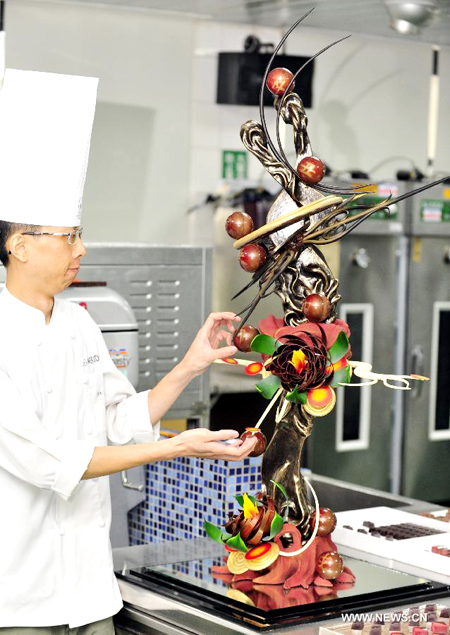In the image, a skilled pastry chef is meticulously fine-tuning a highly ornate food sculpture in a professional kitchen. The slender, bespectacled Asian chef is dressed in a white chef's coat adorned with a logo over the pocket and a name that is not clearly identifiable. He wears a very tall chef's hat, nearly the height of his torso, and khaki pants. The sculpture itself is an extravagant creation that stands approximately four feet tall, crafted to resemble a whimsical, Dr. Seuss-like creature or a fanciful tree with artistic flair. The base of the sculpture is composed of large, decorative chocolate balls and other sweet elements, while the upper part features a twisting structure made from variously shaped lollipops. The design includes swooping horns and vivid red, green, and metallic ornament-like spheres, possibly resembling a festive or Christmas theme. The kitchen backdrop contains stainless steel appliances, trays of chocolate candies, and a blue subway tile outcrop. The bottom right of the image is marked with "www.news.cn," indicating this is a professionally taken photograph.